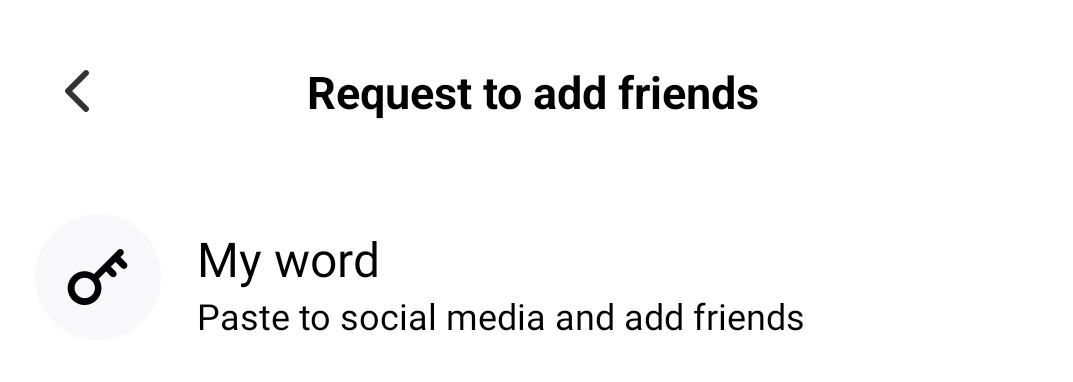This detailed close-up image showcases a user interface screen from an application, specifically focused on a configuration or settings area. Prominently centered at the top is the title "Request to Add Friends." To the left of this title is a left-pointing arrow, presumably for navigation. Below the title, there's a subheading labeled "My Word," accompanied by a key icon situated to its left. Directly beneath the "My Word" section, the screen provides options labeled "Paste to Social Media" and "Add Friends."